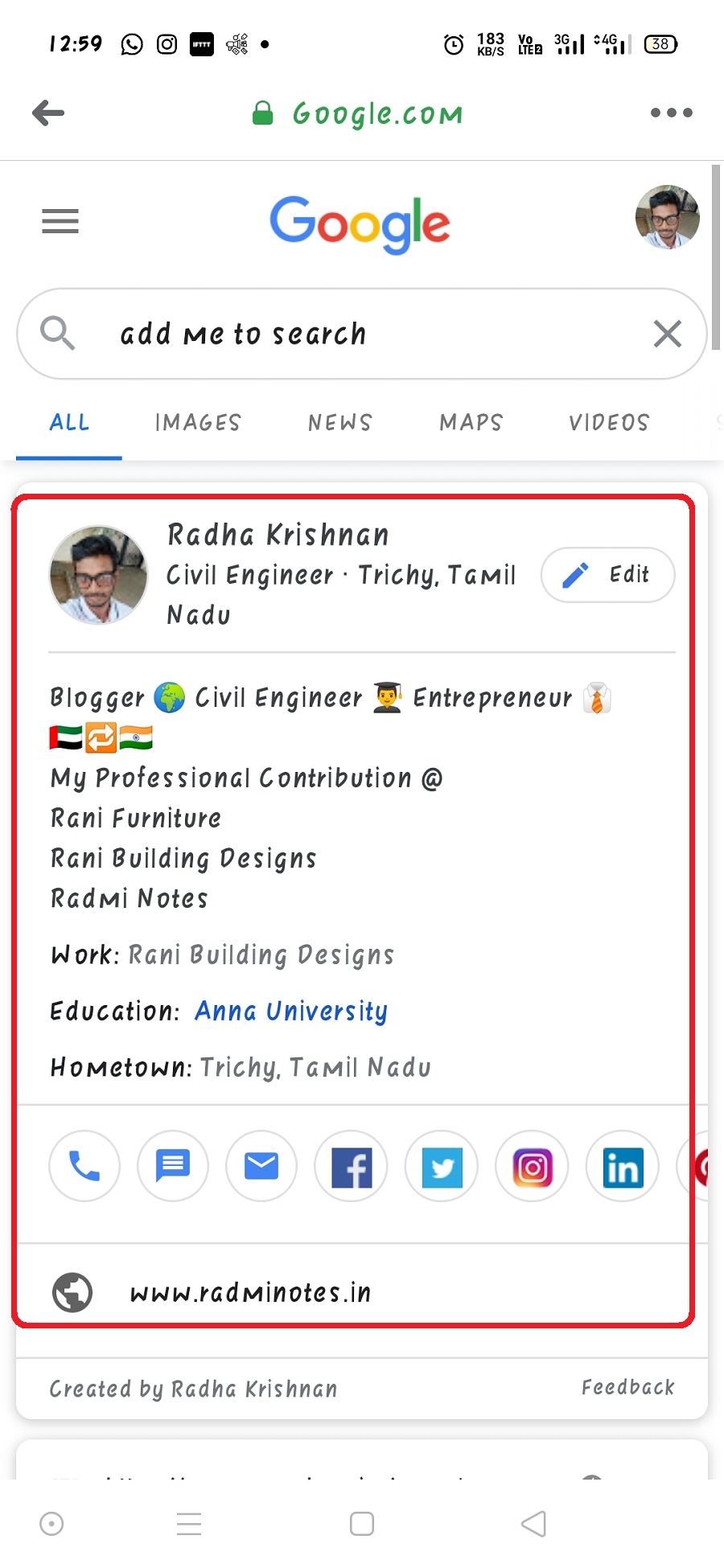In this detailed screenshot of a phone, the background is all white. At the top left corner, "12:59" is displayed in black along with symbols for a phone, Instagram, and a battery percentage icon on the far right, which also indicates connectivity like 3G, 4G, or 5G with full bars.

Centered below this is a green lock symbol typically used for securing doors, accompanied by the text "google.com" in green. To the left of this text is a gray left-pointing arrow, and to the right are three horizontal dots.

Below the "google.com" header is Google's iconic logo in multi-colored letters: a blue "G," a red "O," a yellow "O," another blue "G," a green "L," and a red "E." To the right of these letters is a portrait picture of a gentleman with black hair and glasses of European Caucasian descent, though his face isn't visible.

Below this, there's a cylindrical search bar with rounded edges. Inside this search bar, on the left, is a diagonal magnifying glass icon, and in italicized black text it says, "add me to search."

Below the search bar, the menu items "All," "Images," "News," "Maps," and "Videos" are displayed. "All" is highlighted with a blue underline, while the others are grayed out. 

A red box below these menu items contains a slightly larger, circular portrait of the same gentleman seen earlier. His name, "Raja Krishnan," is written in italicized black text, followed by the title "Civil Engineer" and the tag "Trichy, Tamil Nadu." Next to this information is a diagonal blue pen and the word "edit."

Below this section, there is a thin dividing line, and it lists several roles:
- **Blogger**: with an earth emoji.
- **Civil Engineer**: with a person graduating emoji.
- **Entrepreneur**: with a building emoji.
To the left, flags of India and possibly Palestine are displayed.

In another section titled "My Professional Contribution," it lists projects:
- **Ronnie Furniture**
- **Ronnie Building Designs**
- **Read Me Notes**

Additional information follows:
- **Work**: Ronnie Building Designs
- **Education**: Anna University (highlighted in blue)
- **Hometown**: Trichy, Tamil Nadu (in italicized black text)

At the bottom, icons for Instagram, LinkedIn, Facebook, email, phone, and text are displayed.